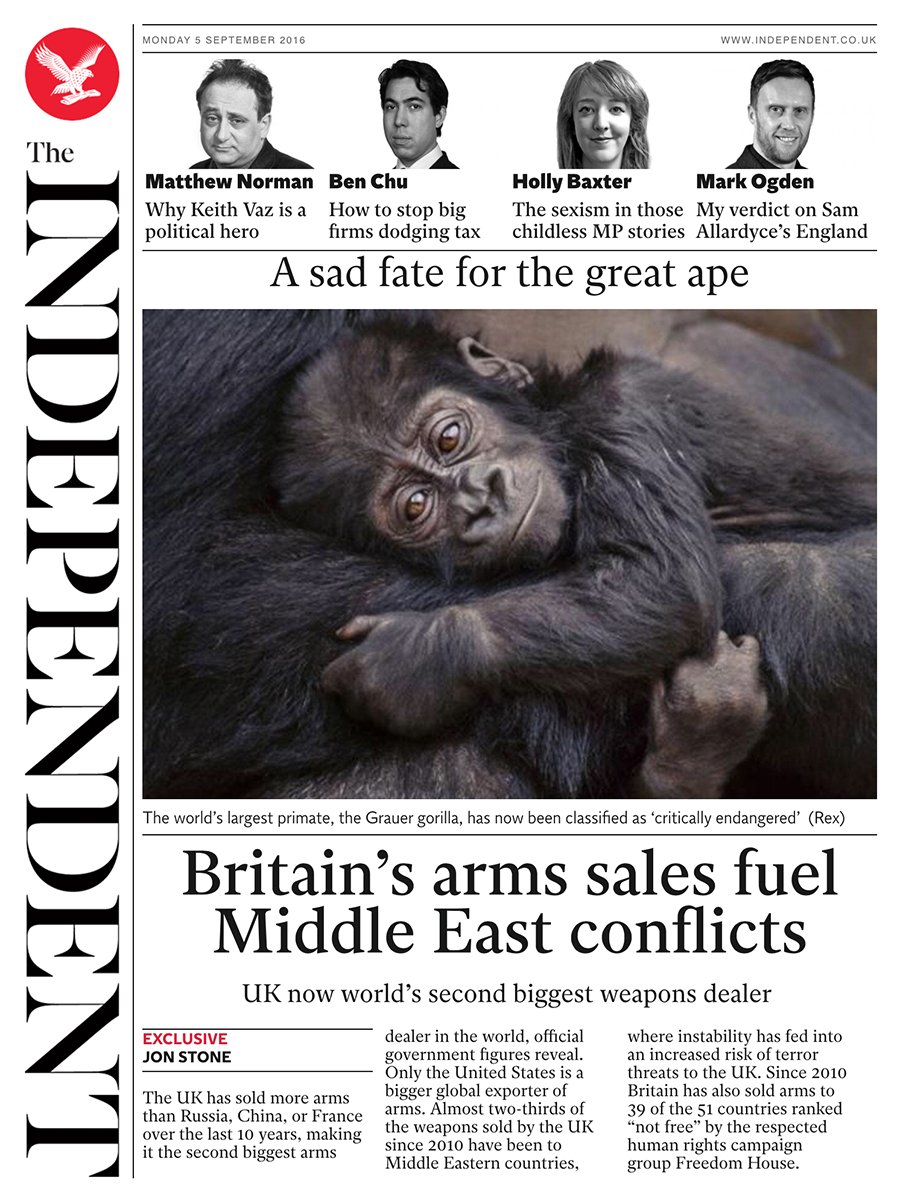A digital edition of The Independent displayed on an unknown device features a prominent banner at the top indicating the publication date as Monday, 5 September 2015, and the web address www.independent.co.uk on the right. The main article, titled "A Sad Fate for the Great Ape," is accompanied by a striking image of an ape. The caption beneath the picture reads: "The World's Largest Primate, the Grauer gorilla, has now been classified as 'critically endangered' (Rex)." The columnist section lists writers Matthew Norman, Ben Chu, Holly Baxter, and Mark Ogden. Another headline beneath the main article states, "Britain's Arms Sales Fuel Middle East Conflicts," revealing that the UK has become the world's second-largest weapons dealer. This exclusive report is authored by John Stone, who is not among the previously listed columnists.